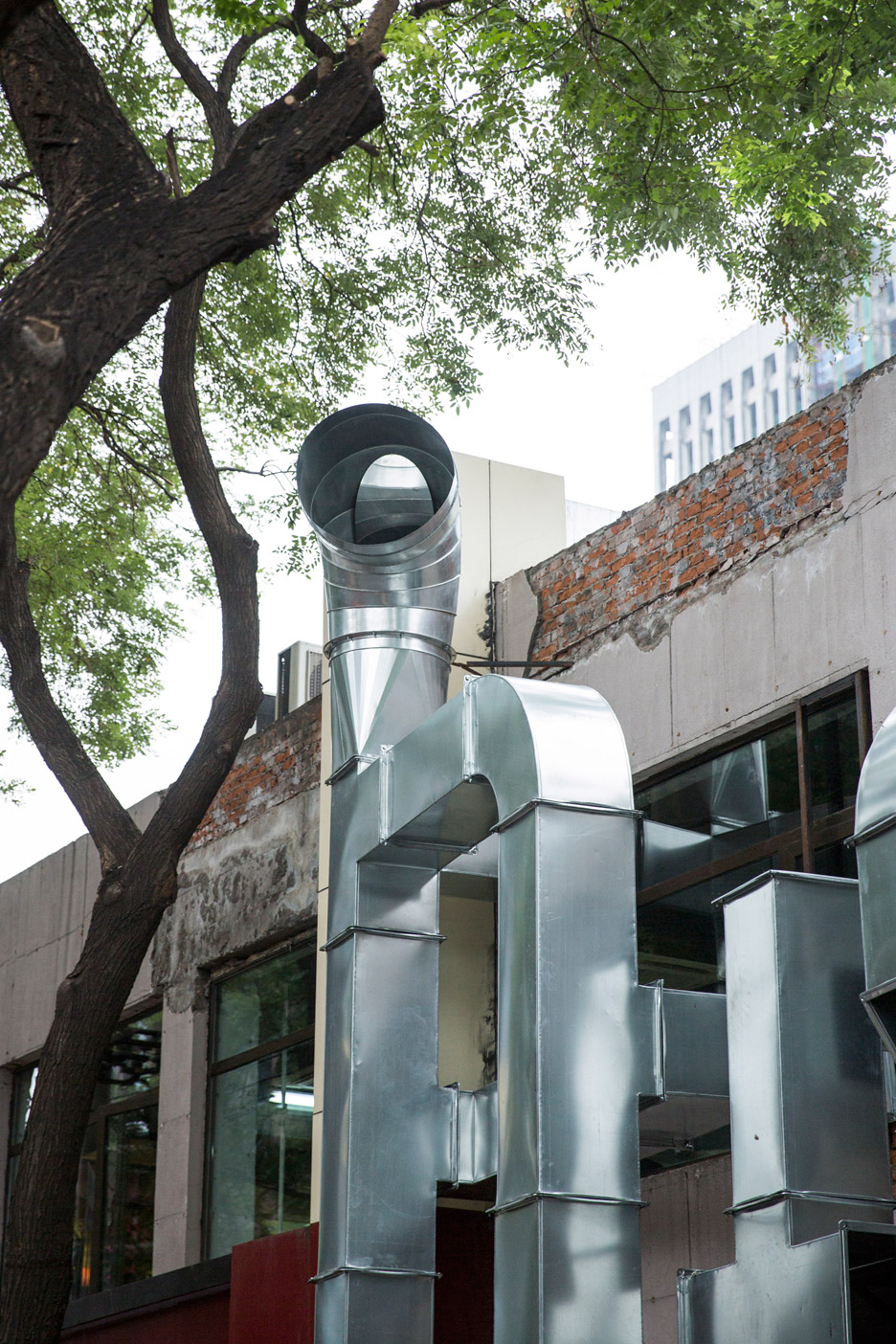The image showcases the exterior of a roughly finished, two-story building that appears to have been refurbished yet retains an exposed brick section near the roof. Below the brick, a row of large windows lines the facade. Prominently featured on the building's exterior is an intricate, art-like installation of HVAC ductwork, composed of rounded and square pieces of galvanized steel, bolted and welded together into an ornate design. In front of this building stands a tree with two trunks and a canopy full of lush green leaves. On the right side of the image, a metal structure, likely an extension of the ductwork, is also visible. Additionally, the top floors of a taller building can be seen in the background, suggesting an urban setting. The scene is captured during daytime, emphasizing the vibrant greenery and the reflective quality of the ductwork.